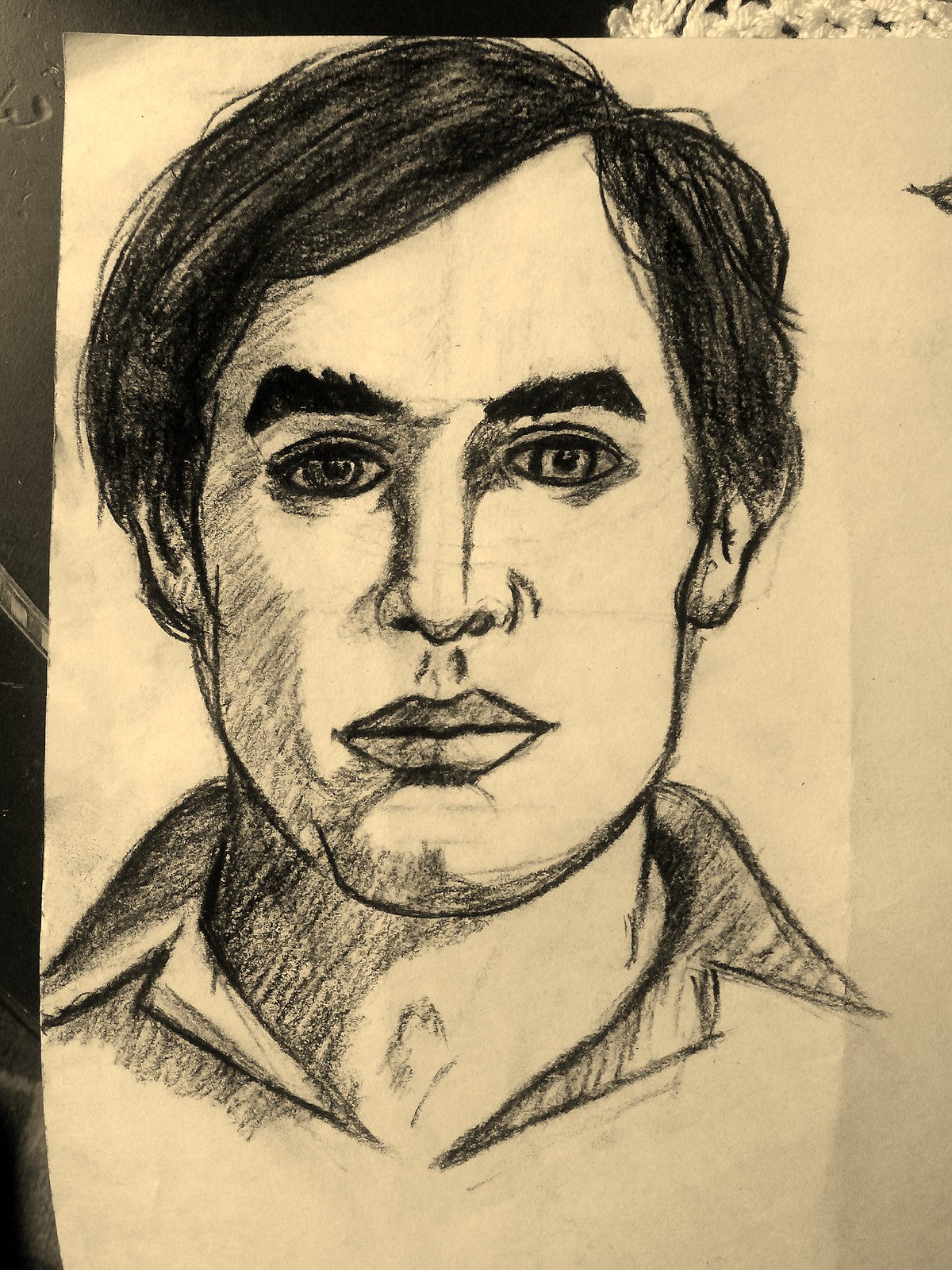A meticulously crafted portrait sketch of a man rendered in a highly realistic style, possibly using charcoal or a dark pencil. The subject displays a contemplative or serious demeanor. His dark hair is artfully swept to the side, exhibiting a slight wave. Well-defined, slightly furrowed eyebrows add to the intensity of his focused gaze. The eyes are strikingly detailed, with clearly visible irises and pupils that suggest deep thought. His facial features include a prominent nose and full lips, with skillful shading accentuating his cheekbones. The structure of his face is rendered with depth and precision, enhancing the three-dimensional quality of the portrait. Subtly sketched, the collar of his shirt further complements the overall mood of introspection that emanates from the artwork.